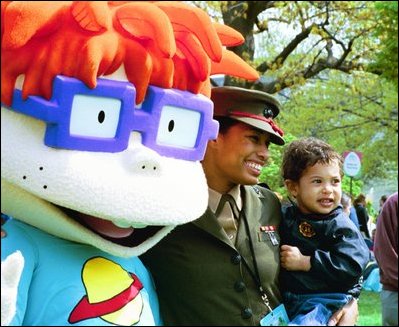In the photograph, a person dressed as Chucky from the Rugrats, identifiable by his red hair, oversized purple glasses, and light blue shirt adorned with a yellow planet and red ring, poses next to a woman in a green army uniform. This woman, smiling warmly, holds a toddler with short brown hair, a blue jacket, and blue jeans. Both the woman and the child are of different skin tones, suggesting the child might be of mixed heritage. The trio is positioned side-by-side, looking at a camera that is just off to the right. In the background, one can see trees, a cloudy sky, and some indistinct figures and limbs of other people, adding to the lively atmosphere that hints this could be an amusement park or similar setting. The large-headed Chucky costume makes a striking visual contrast with the military uniform and adds a whimsical touch to the scene, giving the impression that the photo may have been taken in the early 2000s.